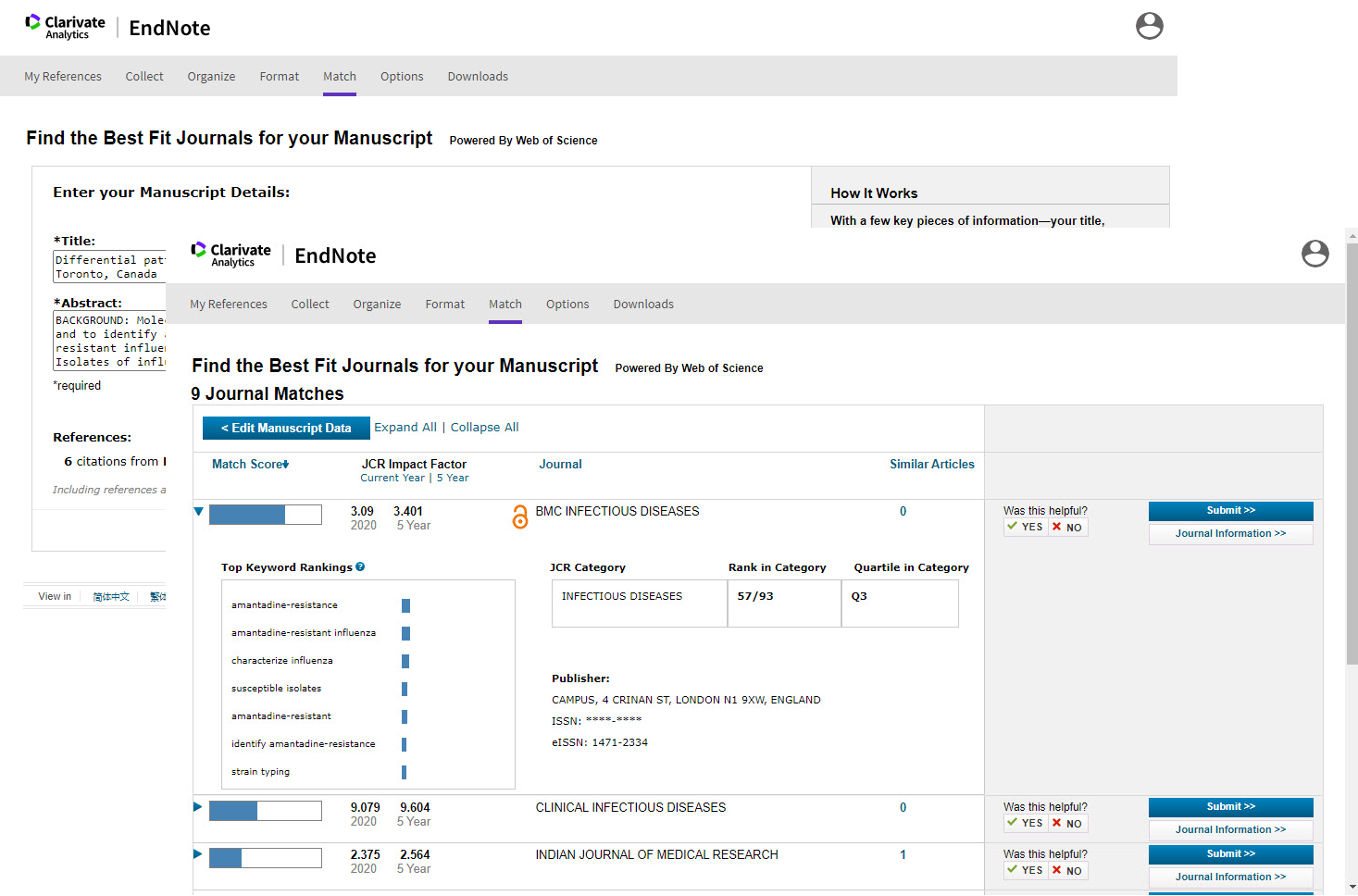The image features a detailed interface of a scholarly tool designed to assist with manuscript management and journal selection, set against a light purple background. 

In the upper left corner, there is a small, black and blue circle bearing the text "Clarivate Analysis" next to "EndNote." A small user icon is also present. Below, a purple box titled "My References" lists the features "Collect, Organize, Format, and Match," with "Match" underlined for emphasis.

A central feature of the screen includes a prominent text box urging users to "Find the best fit journals for your manuscript powered by Web of Science." Below this, a purple outlined box prompts the user to "Enter your manuscript details," specifically requiring "Title" (marked with an asterisk) and "Abstract" (also marked with an asterisk). It highlights these fields as required in reference.

Middle section reiterates "Clarivate Analysis" and "EndNote." The upper right section explains "How it works," indicating that with a few key pieces of information such as your title, you can "Find the best fit journals for your manuscript," presenting nine journal matches. Options to "Edit Manuscript Data" (highlighted in blue with a left arrow) and "Match Search" (highlighted in blue with a down arrow) allow further adjustments.

Further down, several journal listings appear, each with a blue trash can icon for deletion. There are blue arrows pointing right, indicating navigation options. Additional details include the names of journals like "Journal of Infectious Diseases" and categories such as "EMC, Infectious Diseases, Category, Risk Category, Recorded Category, Publisher, and Clinical Infectious Diseases."

On the right side, a large purple box questions "Was this helpful?" followed by a blue checkmark for "Yes" and a red X for "No." Two blue "Submit" buttons appear at the bottom for user feedback.

The interface is rich in functionality, providing users with an intuitive way to manage and match their manuscripts with suitable academic journals.